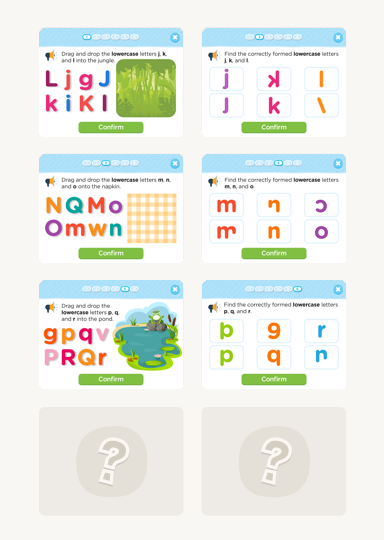The image depicts a learning application interface, featuring two columns of four square mini windows each. The windows contain various interactive elements designed for educational purposes. 

In the first column, the top three squares each display an alphabet-themed activity colored differently for visual distinction. These squares have a small green "Confirm" button and a red "X" icon in the top corner. The first square instructs users to "drag and drop the lowercase letters J, K, and L into the jungle," accompanied by an illustration of a jungle. The second square asks users to "drag and drop the lowercase letters M, N, and O into the napkin," featuring an image of a napkin as the drop target.

The fourth square in the first column, as well as all four squares in the second column, do not display similar content. Instead, these squares are gray with a circle containing a question mark in the center. This suggests that the activities or content for these squares may not be loaded or are inactive.

Overall, the interface appears to be part of an educational application aimed at helping users, likely children, learn and practice the alphabet through interactive drag-and-drop activities.